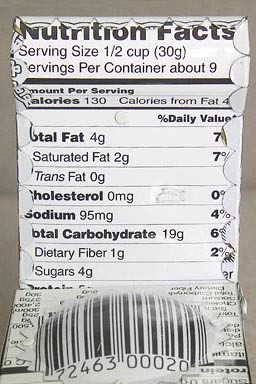This colour photograph presents a detailed close-up of a nutritional label against a beige background that might be perceived as greyish-brown. The label itself is predominantly white with black text. At the top, it prominently features the heading "Nutrition Facts" followed by detailed information including a serving size of half a cup (30 grams) and approximately nine servings per container. Below, the label lists various nutritional details: 130 calories per serving, 4 grams of total fat, 0 grams of cholesterol, 95 milligrams of sodium, and 19 grams of total carbohydrates.

This nutritional label is positioned vertically and is overlapped at the bottom by another label placed horizontally, forming a right angle. The second label, which is similar in appearance, includes a prominently displayed UPC barcode. This barcode appears bubbled up or curved, suggesting it might be attached to a plastic or metal surface molded into a dome shape with zigzag-cut edges. The barcode-segment appears to be folded or bunched at the middle, contributing to its curved appearance, and is affixed below the main nutritional label. The entire setup almost looks like a deliberate arrangement, with the nutritional facts label and the barcode displayed together against the soft-hued background, giving an impression that someone might be collecting these labels.